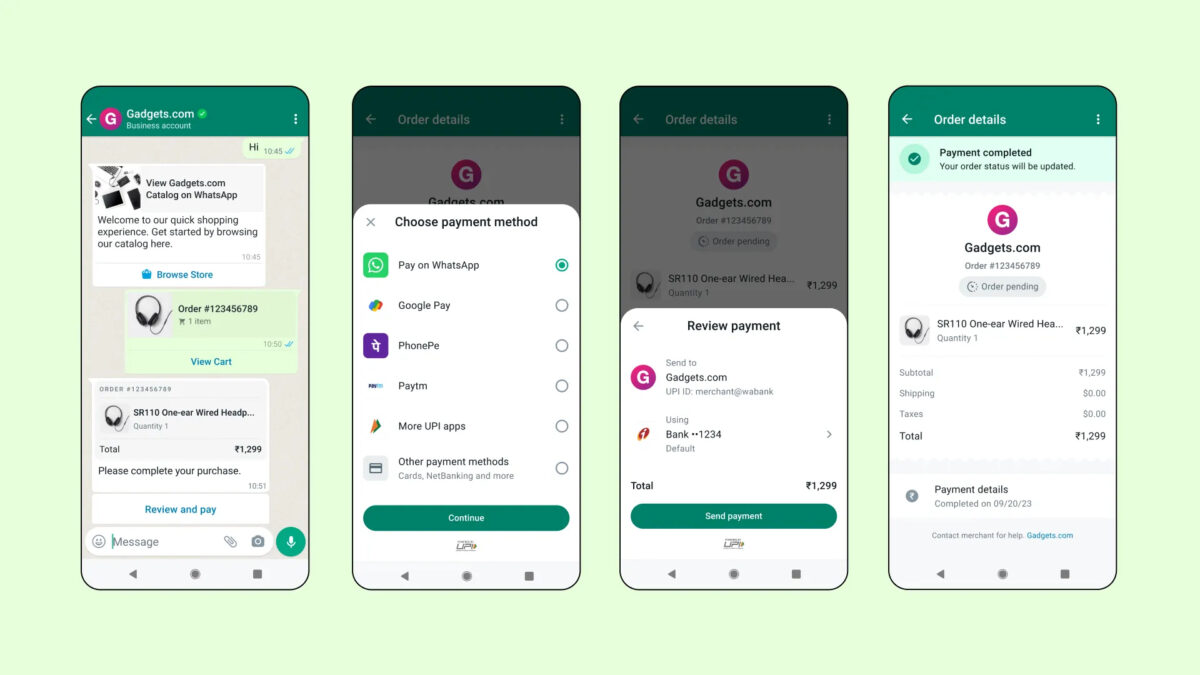The image displays four sequential screens depicting the purchasing process on Gadgets.com via WhatsApp. 

1. **First Screen (Leftmost)**: This screen features a white 'G' inside a pink circle at the top, with the title "Gadgets.com". Below it, a message reads "View Gadgets.com catalog on WhatsApp. Welcome to our quick shopping experience. Get started by browsing our catalog here." An order number "1, 2, 3, 4, 5, 6, 7, 8, 9" is shown. A headset is pictured with the text "View Cart" below it. The headset is priced at $1,299. It instructs users to "Please complete your purchase, review, and pay."

2. **Second Screen**: This panel prompts the user to "Choose payment method." Various payment options are listed, including Google Pay, PhonePe, Paytm, more UPI apps, and other payment methods. At the bottom, there's a "Continue" button.

3. **Third Screen**: This screen is a payment review for Gadgets.com, showing a bank card with the partial number "1, 2, 3, 4". A button labeled "Send Payment" is visible.

4. **Final Screen (Rightmost)**: The screen confirms that the payment has been completed on Gadgets.com. The breakdown includes a subtotal of $1,299, with zero shipping and taxes, making the total $1,299. The payment was completed on 04/24/23.

This sequence effectively walks the customer through the steps of browsing, selecting a payment method, reviewing the payment, and receiving confirmation of their purchase.